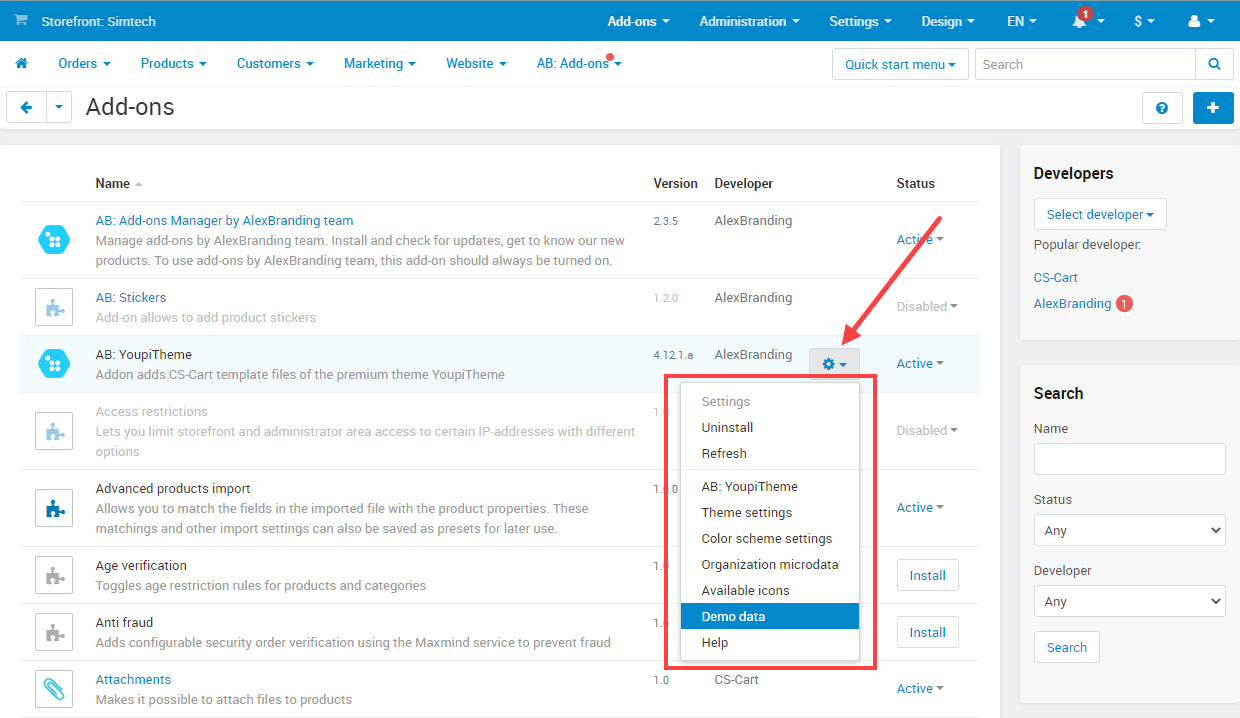This is a detailed screenshot of a web page displaying the interface of an online storefront platform, identified by a blue bar at the top with "Storefront Centech" or possibly "SunTech." Directly beneath this blue bar is a submenu featuring tabs labeled "Orders," "Products," "Customers," "Marketing," "Website," and "AV Add-ons," with the "Add-ons" tab currently selected. 

Below this submenu, the page is organized into a table with columns for "Name," "Version," "Developer," and "Status," although the text is notably small and somewhat difficult to read. Within this Add-ons section, the table lists nine distinct items available for use. The specific Add-on titled "AB: U Theme" is prominently circled in red, drawing attention to its selection.